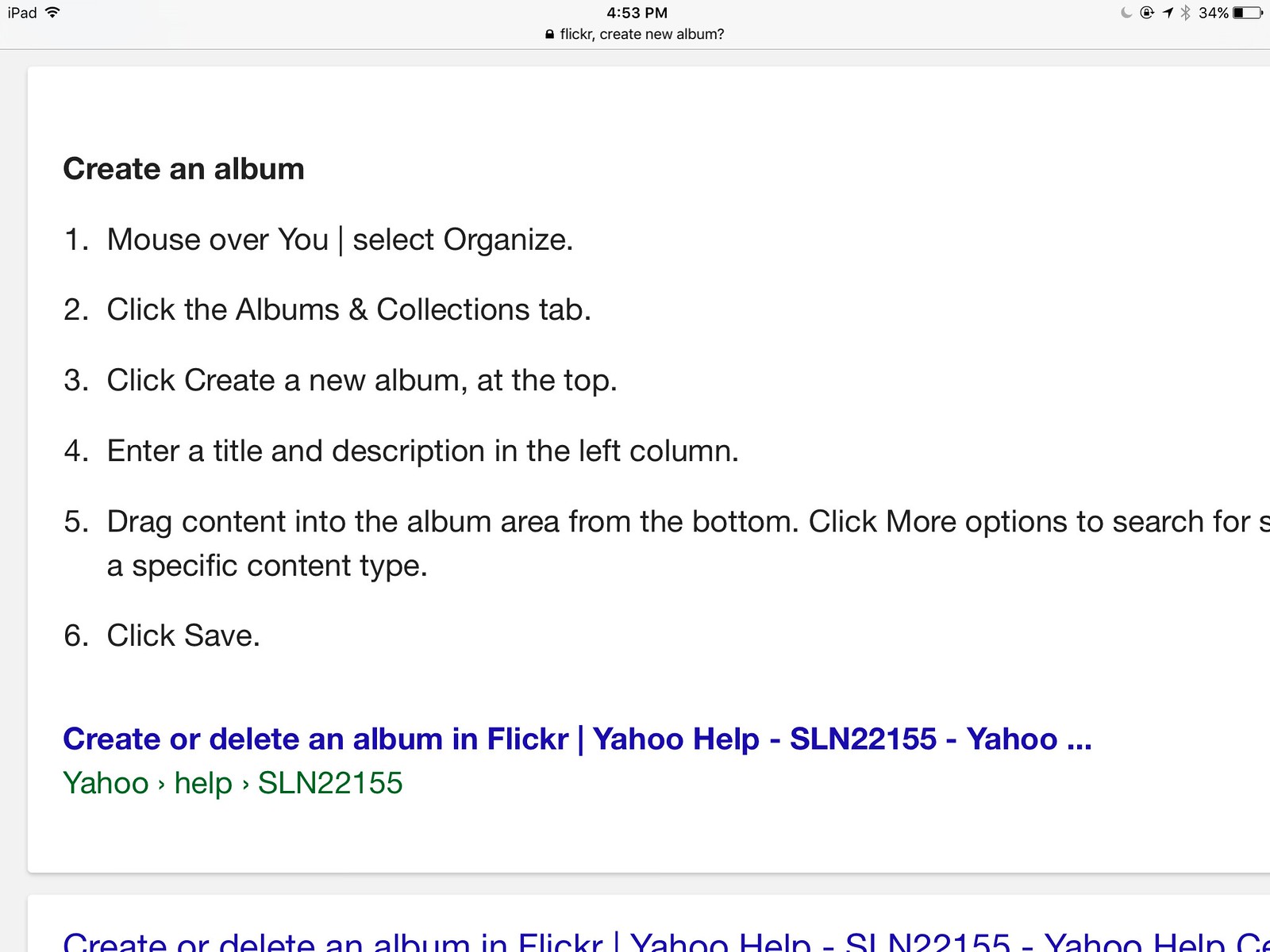The image is a screenshot from an iPad displaying step-by-step instructions for creating an album on Flickr. At the top, the device status indicators such as the time, battery sign, and percentage are visible. The instructions are listed against a white background with black text. They are as follows:

1. Move the mouse over "You" and select "Organize."
2. Click the "Albums and Collections" tab.
3. Click "Create a New Album" at the top.
4. Enter a title and description in the left column.
5. Drag content into the album area from the bottom. Click "More Options" to search for a specific content type.
6. Click "Save."

Below the instructions, in blue text, it says "Create or delete an album in Flickr, Yahoo help, S-L-N-2-2-1-5-5 Yahoo." In green text, it repeats "Yahoo help, S-L-N-2-2-1-5-5 Yahoo." There is additional text at the bottom of the screenshot, but it is cut off.